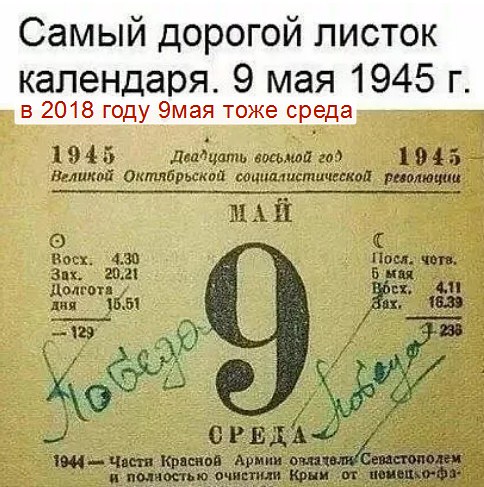The image depicts a worn, grainy photograph of a Russian document dated March 9, 1945. The document appears to feature a mixture of printed and handwritten text in Russian, with notable emphasis on historical references. The headline, when translated to English, reads "The Most Expensive Piece of the Calendar, May 9, 1945." Throughout the document, the date of May 9, 1945, is highlighted as significant, noting that in 2018, this date fell on a Wednesday. The text references the 28th year of the Great October Socialist Revolution. Additionally, it commemorates the capture of Sevastopol by units of the Red Army in 1944 and the complete clearing of the Crimea of the Pemets. The central portion of the document prominently features a large, bold number "9" and further includes numbers such as 1944 and 1945, with additional handwritten annotations in green ink. The overall appearance of the document suggests it might have been excerpted from a textbook, featuring a cream-brown background with red and black text, underscored by lines of foreign text both printed and in cursive handwriting.